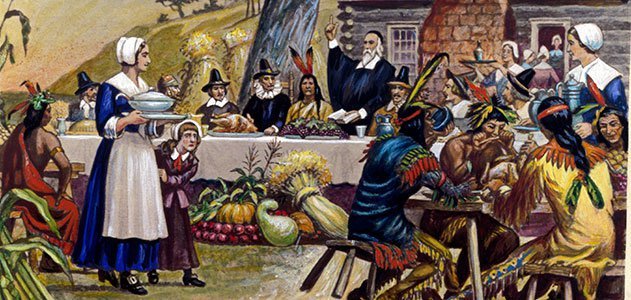The image depicts a detailed 19th-century illustration of the first Thanksgiving feast shared between the Native Americans and Pilgrims. In the foreground, a pilgrim woman dressed in a blue dress with a white apron and bonnet holds a silver tureen. Beside her, a young girl peers shyly from behind her skirts. To her left, four Native Americans in traditional garb, adorned with feathers, are seated at a separate table, engaged in eating. Notably, one wears a distinct blue, red, and green outfit, another is clad in yellow with orange feathering and detailed designs, a bare-chested man is biting into a piece of meat, and another face is partially visible.

At the center of the image is a long table draped with a white tablecloth, hosting a gathering of Pilgrims and Native Americans. A prominent pilgrim man with a long white beard stands, holding a book (possibly a Bible) and raising two fingers in the air. Behind the main table, a log cabin with a brick chimney stands against a backdrop of rolling green hills and trees, suggesting a tranquil, late-afternoon setting with a yellow and orange sky indicating sunset.

In the background, you can see various activities and elements: a woman pilgrim exiting a house, another carrying a bottle of water, and a collection of cornstalks, vegetables, pumpkins, gourds, and haystacks spread across the ground. The overall setting captures the festive and communal spirit of this historic gathering, highlighting the blending of cultures and the sharing of a bountiful harvest.